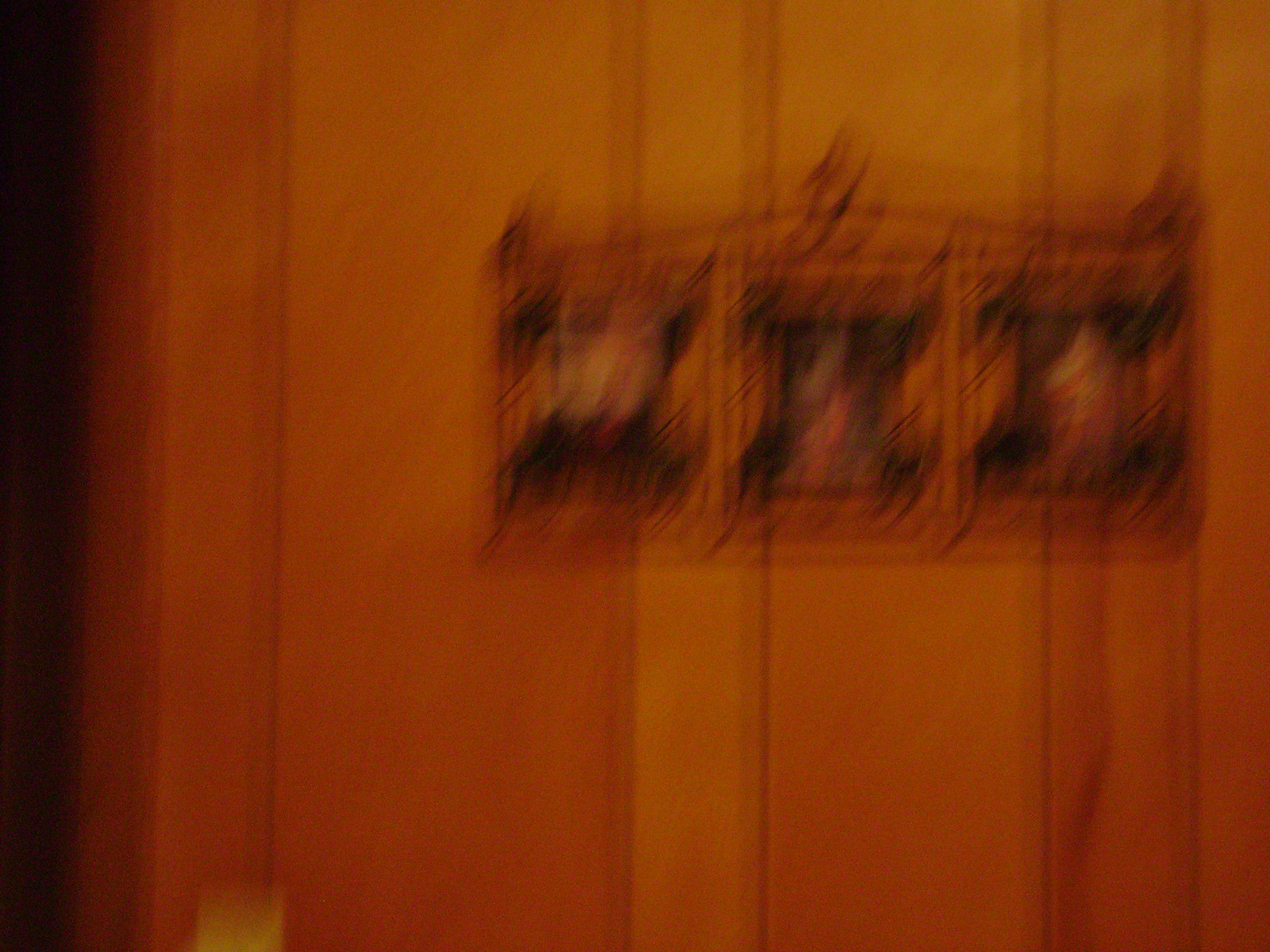The image showcases a wall that appears to be a blend of brown and reddish hues. Vertical black lines run down the surface, creating a rhythmic pattern. Positioned on the wall is a blurry, black-outlined square, seemingly hanging by a cord visibly extending from the top. The inner design of the hanging square features three smaller squares, each filled with progressively darker shades of black, forming an "X" pattern with the corners missing. Among these, the central square is notably more solid in color. To the far left of the central design is another section that is predominantly solid black, occupying about a sixteenth of the total visible area. Additionally, a small, blurry yellow square is noticeable at the bottom right. Furthermore, black lines are also apparent on the hanging piece, adding to its intricate design.